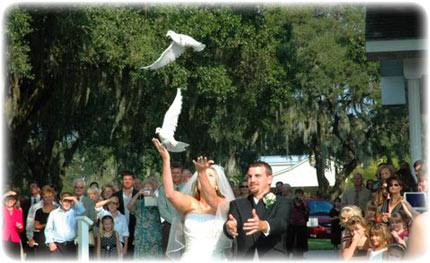This horizontally rectangular wedding photograph, with softly fading rounded borders into a white background, captures a joyous moment as two white doves are being released by the newly married couple. The couple is front and center, bathed in bright sunlight against an outdoor backdrop. The bride, a white woman with blonde hair, stands on the left wearing a white wedding dress and veil. Her arms are triumphantly raised above her head. On her right, the groom, a white man with short-trimmed brown hair and a goatee, is dressed in a black tuxedo adorned with a white flower on his lapel. His hands are open and extended in front of him. Above them, the white doves soar upwards. In the background, there are elegant green willow tree branches hanging down, and to the right, part of a white house with a pillar is visible next to a red car. A crowd of wedding guests of various ages and formal attire watches the spectacle, many shielding their eyes from the bright, warm sunlight.